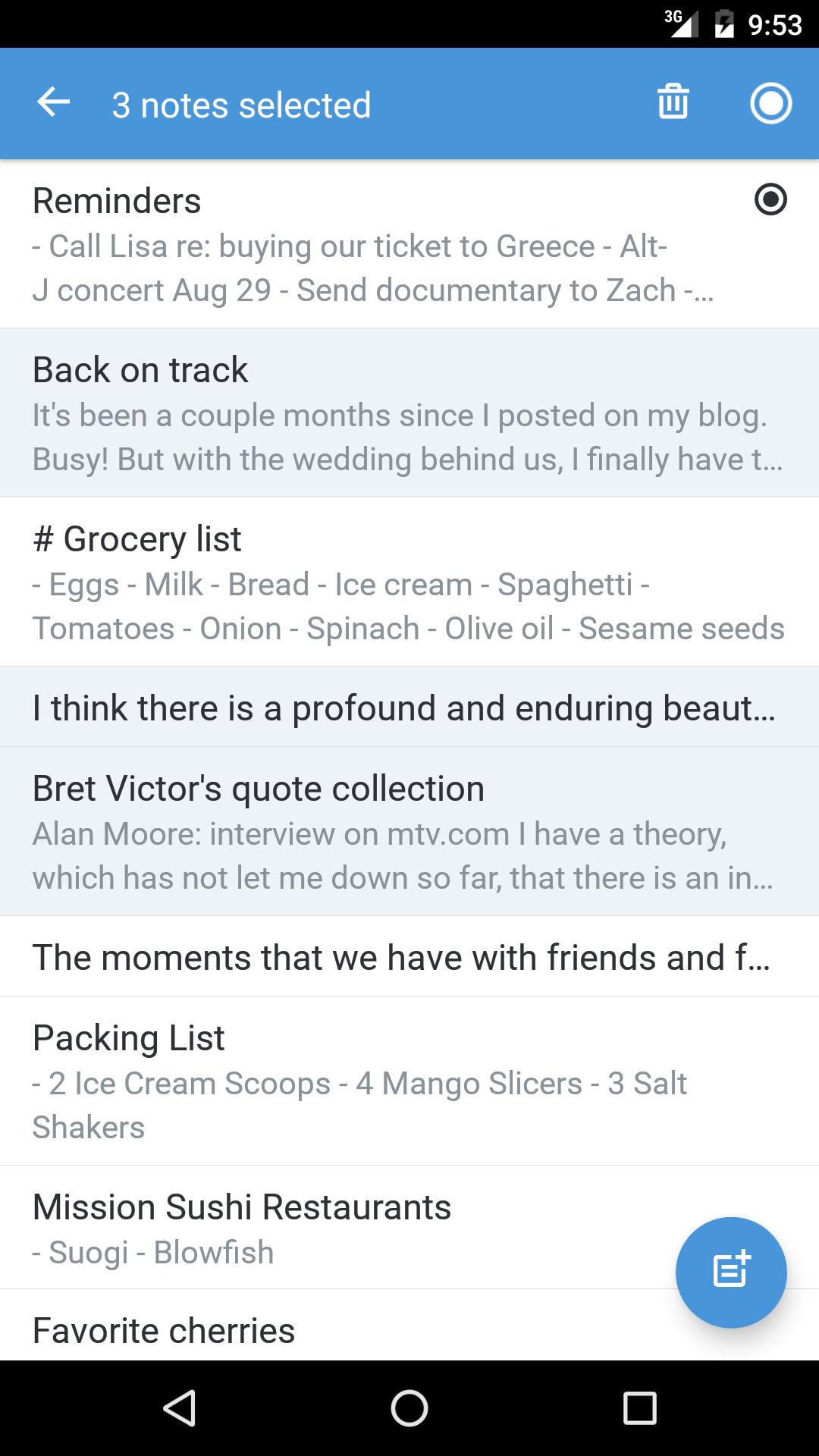The image is a screenshot of a notes app, likely taken on an Android device. At the top right of the screenshot, various status icons are visible, including a "3G" network indicator, a battery charging icon, and the current time displayed as 9:53. Below these status icons, the app interface shows that three notes are selected. 

The list of selected notes, with visible titles, is as follows:
1. **Reminders**
2. **Back on Track**
3. **Grocery List** (preceded by a pound symbol)
4. A note titled "A profound and enduring…” (the rest of the title appears to be cut off, potentially finishing with "beauty")
5. **Brett Victor's Quote Collection**
6. **The Moments That We Have Friends** (the rest of the title is cut off)
7. **Packing List**
8. **Mission Sushi Restaurants**
9. **Favorite Cherries**

This organized overview provides a structured glimpse into the content and titles of the notes within the app.